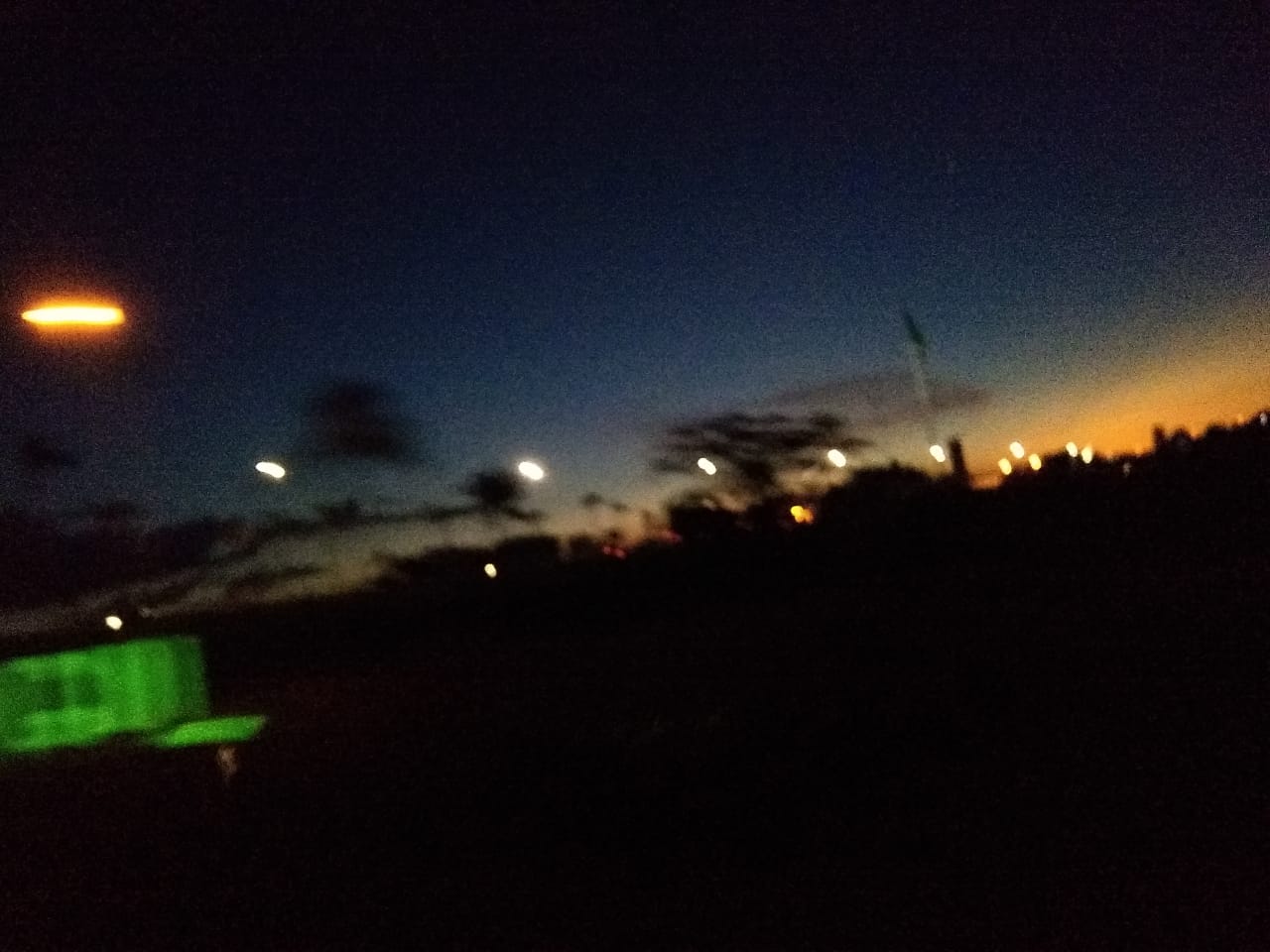This photograph captures a blurry, low-resolution nighttime outdoor scene, likely taken around dusk or sunset. The sky transitions from a dark black at the top to a deep navy blue, and then to shades of medium blue and orange-yellow near the horizon. The sun appears to be setting, casting an ethereal glow on the silhouetted trees and buildings scattered across the background. To the left, there's a distinct bright orange light, likely from a lamppost, adding a warm contrast to the scene. In the bottom left foreground, there is a luminous lime-green rectangular object, potentially a dumpster or a train car, though the haziness obscures its exact details. The scene is dotted with what appear to be street lights or other illuminating sources, providing faint highlights against the dusky landscape.